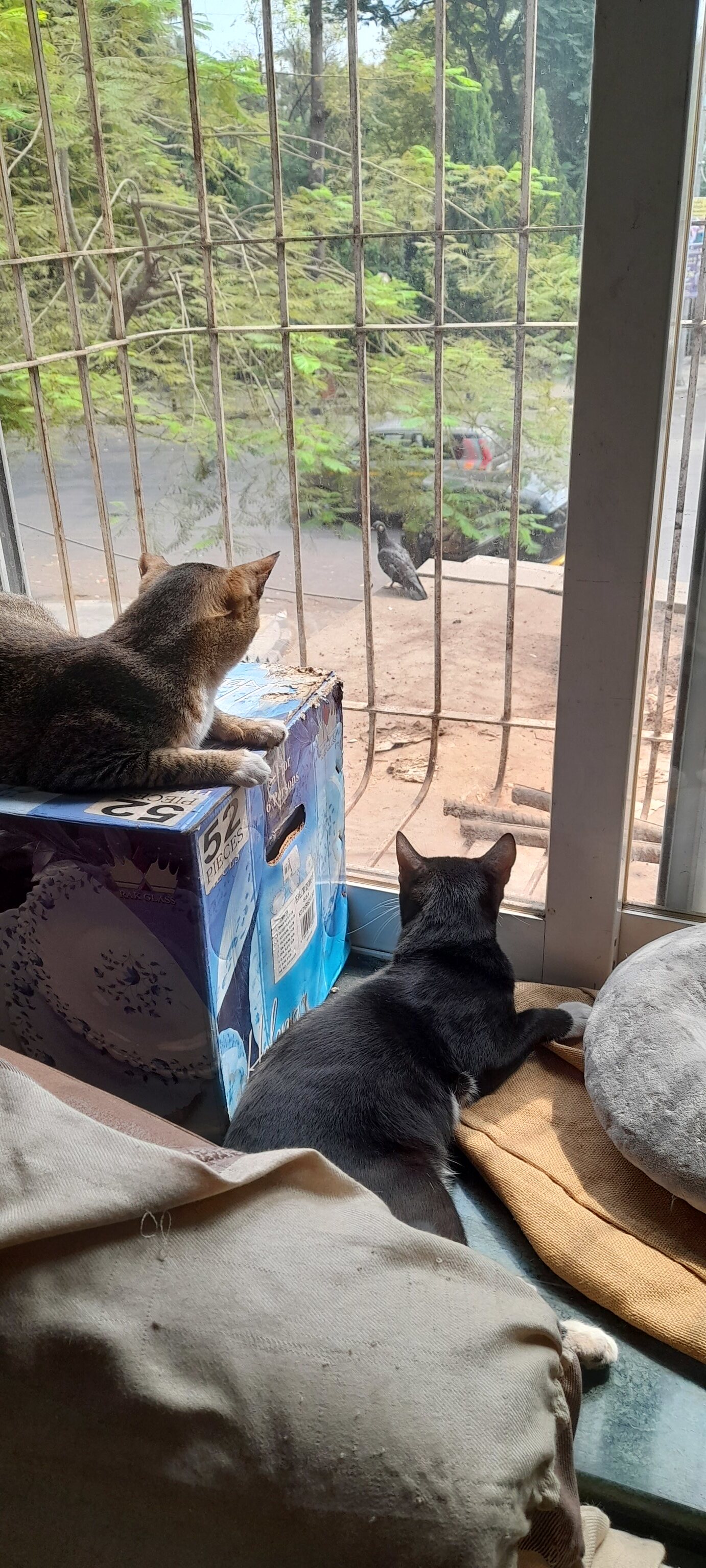Inside a cozy room, we see a scene depicting two cats intently gazing outside through a large window. The bottom half of the image shows the room's interior, where a black cat with a white paw lies at the center, while a brown cat with dark brown and black fur perches on a light and dark blue box with the text "52 pieces." Below them rest gray and tan blankets scattered on the floor. 

The upper half of the image captures the view outside the window. The window is framed by white metal bars, resembling either protective bars or part of a cage structure. Outside, a gray bird stands on a dirt windowsill, watched eagerly by the cats. To the left, tree branches with light green leaves frame the top of the scene, while a distant road and some hidden, possibly water-like feature or forest can be seen in the background. The setting vividly contrasts the comfort of the indoor space with the natural elements outside, highlighting the cats' attention to the bird beyond the fence and trees.